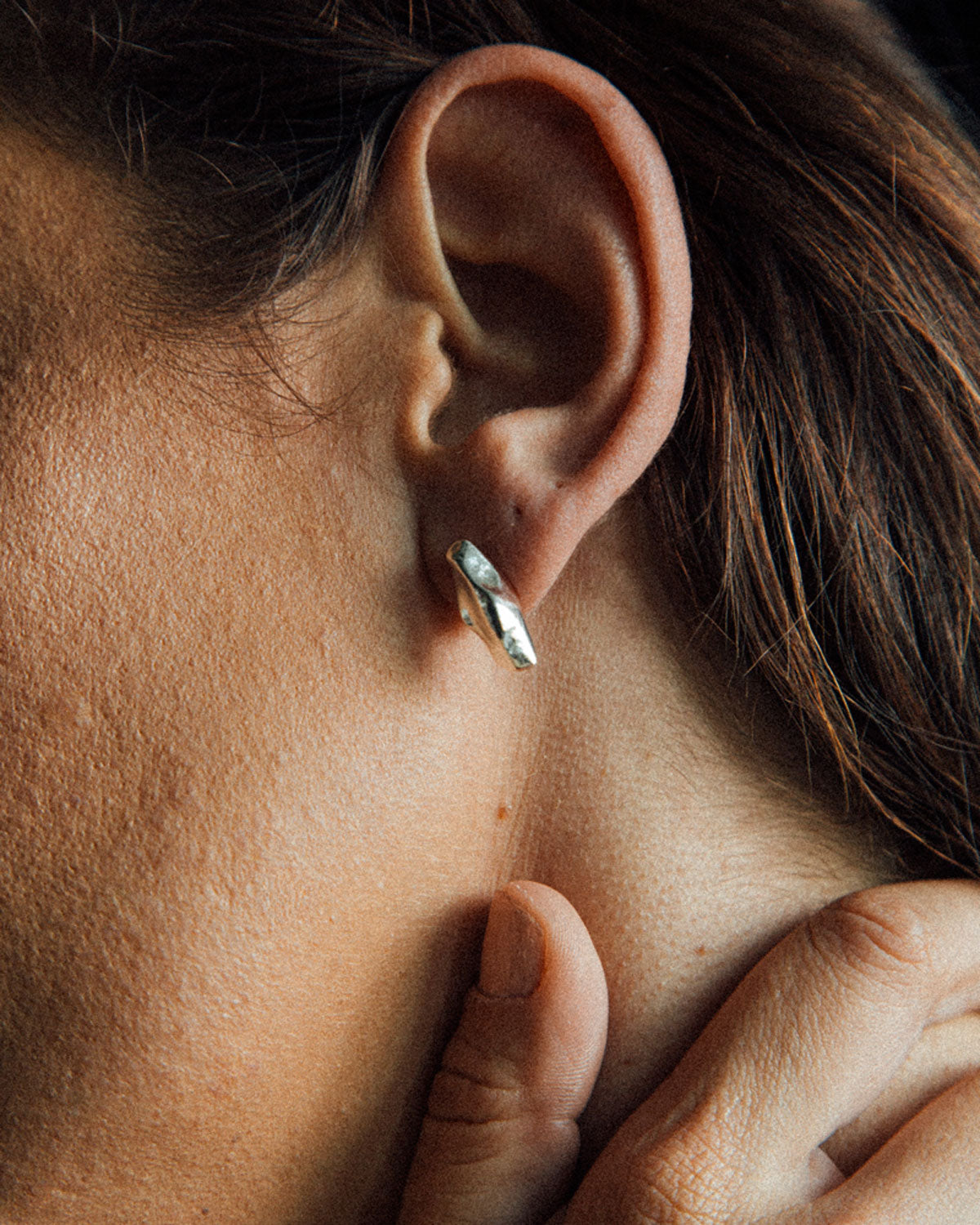This close-up, portrait-mode image prominently features the ear and hair of a Caucasian individual, presumed to be a woman given the overall context. The person's light brown hair is neatly tucked behind the ear, cascading down the neck. The ear showcases an earring made of metal, described as a very small, thin piece of jewelry, along with two additional piercing holes above it that currently have no earrings. Below the ear, a hand is visible resting on the neck, with the thumb, index finger, and a glimpse of the middle finger apparent. The skin tone of the hand matches that of the ear, emphasizing a consistent, light complexion. The image focuses on these details, with no visible indication of the person's eyes or mouth.